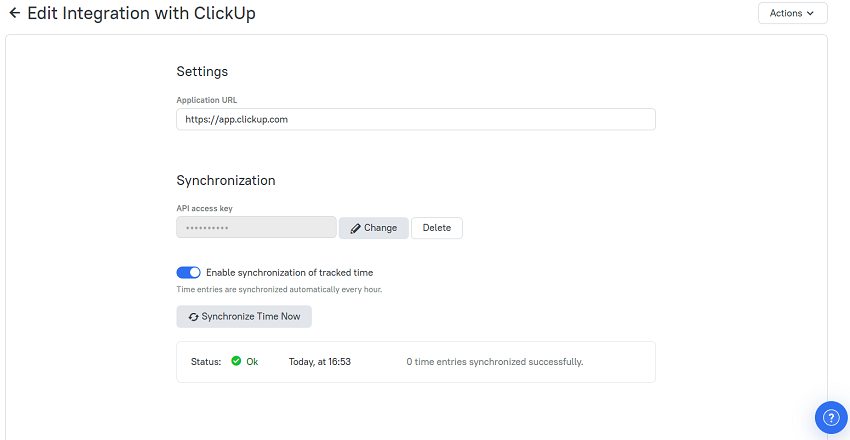This image is a screenshot of a ClickUp web page, a software tool used for project management. The background of the page is white. At the top left, written in dark gray font, is "Edit Integration with ClickUp," with "ClickUp" being styled with a capital 'C' and a capital 'U'. To the left of the word "Edit," there is a left-pointing arrow icon.

On the far right side of this top section, there's a gray-outlined rectangle containing the word "Actions" accompanied by a downward-pointing arrow, indicating a dropdown menu. Just below this top section, there is a very light gray horizontal line.

Underneath this line, the word "Settings" appears in gray font, followed by "Application URL" with an input field displaying "https://app.clickup.com". Below this, there is a section labeled "Synchronization." In this section, above a gray rectangle, there is the label "API Access Key." The actual key is obscured by dots for security. To the right of this key, there’s a gray rectangle with the word "Change" and a small pencil icon. Further right, another rectangle, this time white, bears the word "Delete."

Beneath this, there is a blue button labeled "Enable synchronization of tracked time." In smaller print below this button, the text reads "Time entries are synchronized automatically every hour." Another gray rectangle follows, carrying the label "Synchronize time now" in gray font.

Adjacent to this, a white rectangle displays the word "Status," followed by a green circle with a white checkmark inside it, and the word "OK." To the right, it notes the time "Today at 16:53," and indicates that "Zero time entries synchronized successfully."

Finally, in the lower right-hand corner of the screenshot, there is a blue circle featuring a white question mark.